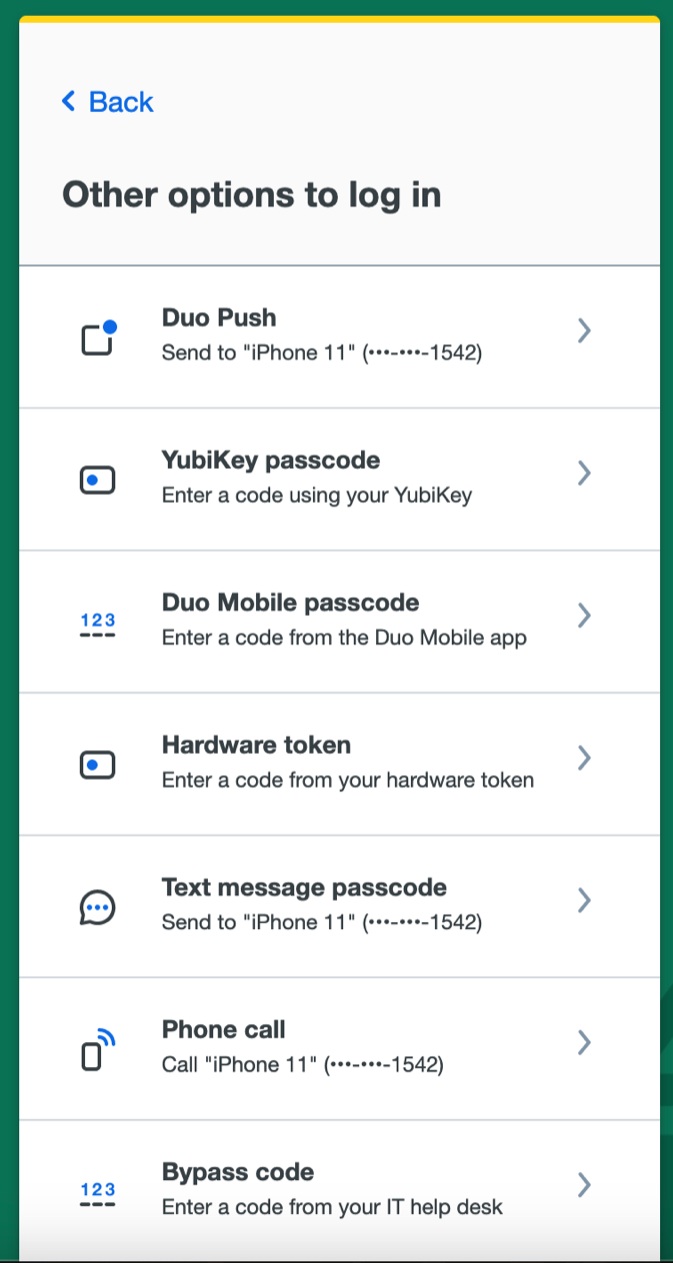This image is a screenshot taken from a phone. The screen displays a login interface, characterized by its vivid colors and detailed options. Encircling most of the screen is a green border that surrounds the sides and top but stops short at the bottom. Just inside the green border at the top is a yellow line that runs horizontally but does not extend down the sides or bottom.

At the top left of the screen is a blue button labeled "Back." Below this, the interface lists various options to log in, each delineated in its own section with a right-facing arrow (a sideways gray "V") at the end.

The options are as follows:

1. **Duo Push:** Sends a push notification to the iPhone.
2. **YubiKey Passcode:** Prompts to enter a code using a YubiKey.
3. **Duo Mobile Passcode:** Requires a code from the Duo Mobile app.
4. **Hardware Token:** Requests a code from a hardware token.
5. **Text Message Passcode:** Sends a passcode via text message to an iPhone 11, displaying only the last four digits of the phone number.
6. **Phone Call:** Initiates a call to the iPhone 11, again showing only the last four digits of the number.
7. **Bypass Code:** Asks for a code provided by the IT helpdesk.

Each option is presented clearly with explanatory text, ensuring users understand how to proceed with their login.